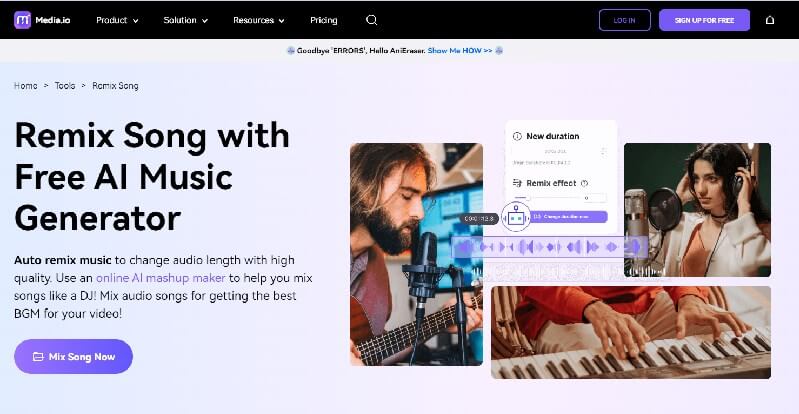The image depicts a webpage dedicated to musicians and music creators, branded under the "MediaIA" logo prominently displayed at the top. The header features navigational elements, including "Product," "Solution," and "Resources," each accompanied by a drop-down arrow, followed by "Pricing" and a search icon resembling an hourglass. To the far right, there are two buttons: "Log In," enclosed in a black-background square, and "Sign Up for Free," highlighted in a blue-background square. 

The background of the page is light blue, with the text "Goodbye errors, hello, anti..." (the remaining text is blurry and unclear, possibly "anti-error") prominently displayed. Below this slogan is a blue hyperlink labeled "Show me how." Further down, there are additional navigation options: "Home," "Tools," and "Remix Song."

The focal point of the page highlights in bold black letters: "Remix Song with Free AI Music Generator." Underneath this headline, descriptive text explains: "Auto-remix music to change audio length with high quality. Use an online AI mashup maker to help you mix songs like a DJ. Mix audio songs for getting the best BGM for your video." The words "online AI mashup maker" serve as a hyperlink.

Next, a blue oval button with white text urges users to "Mix Song Now." To the right, there are images showcasing various individuals engaged in music creation: 

- The person on the left holds a guitar and sings into a microphone. He has a thick brown beard, mustache, and wispy long brown hair.
- In the middle, a message pertains to "new duration and remix effect," though the rest is unclear, likely detailing the functionality of the remix AI generator.
- To the right, a female musician wears headphones and is poised to sing into a microphone. She is dressed in a long-sleeve open jacket with an orange top underneath.
- At the bottom, a person plays the piano, dressed in a long-sleeve shirt and khaki pants.

The images and text collectively convey how users can leverage the AI-powered tools to enhance and mix their music effortlessly.